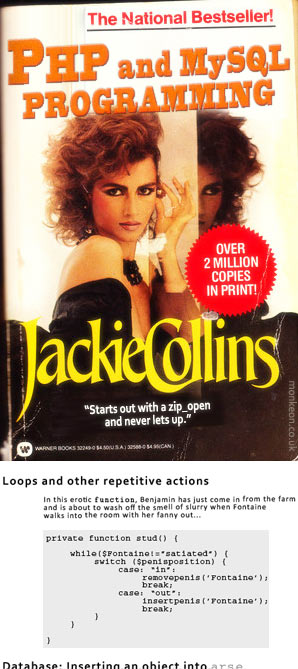Certainly! Here is a detailed descriptive caption for the image:

"An intriguing and whimsical cover of either a book or a DVD titled 'PHP and MySQL Programming.' The headline 'National Bestseller!' is prominently featured in bold, red text, underlined with a thick black line. The title 'PHP and MySQL Programming' appears in a striking orange font. The cover design takes a tongue-in-cheek approach, juxtaposing programming themes with a fashion model motif. The model, with flowing reddish-brown hair and a provocative look, gazes directly at the camera. She is dressed in an elegant black formal dress, evoking a sense of glamour.

The author's name, Jackie Collins, is displayed in a vibrant Sanskrit yellow font along the bottom middle of the cover. Below the author's name, a quote reads, 'Starts out with a zip and never lets up.' Towards the center-right, a red award-like button with frilled edges declares, 'Over Two Million Copies in Print,' written in white text.

On the lower portion of the cover, against a white background, is the text 'Loops and Other Repetitive Actions.' Beneath this, a subtext reads, 'In this erotic function, Benjamin has just come in from the farm and is about to wash off the smell of slurry when Fontaine walks into the room with her fanny out.' Overlaying a dark gray background box, a block of pseudocode defines a private function:

'private function stud() {
    while ($Fontaine != satiated) {
        switch (position) {
            case ‘Remove_Venus’:
                $Fontaine->break;
            case ‘Insert_Venus’:
                $Fontaine->break;
        }
    }
}'
The last line of this function appears to be cut off, adding an element of intrigue and continuity."